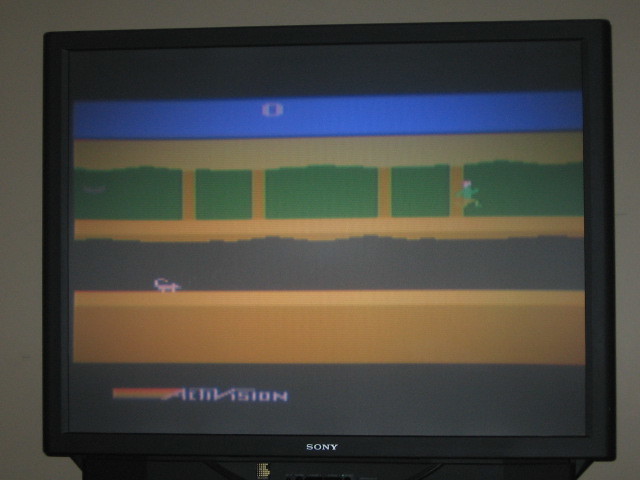This photo captures an old, square-shaped Sony television prominently displaying an 8-bit video game. The Sony logo can be seen at the very bottom of the TV screen. The game in question appears to be published by Activision, as indicated by the text at the bottom of the display. The screen is divided into multiple horizontal bands, with the topmost band featuring a blue background, possibly depicting the sky, and a central symbol that might represent a zero or a sun. Below this is a band of green pixels suggesting a level of trees or grass. Within this green section, a pixelated figure of a man is seen running. The lowest band, representing an underground section beneath the trees, is colored brown and contains a small, pinkish creature resembling a scorpion. The image evokes nostalgia for retro gaming and the early era of pixel art.